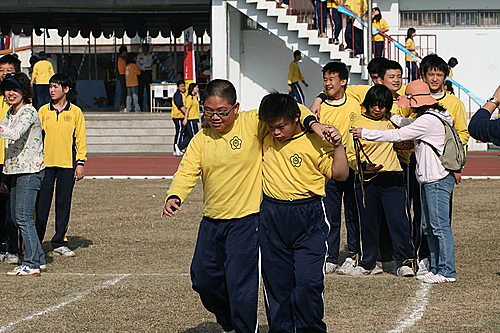In this outdoor image, a group of children is gathered on a ground that appears to be covered either in gravel or short, brown grass. The exact composition of the ground remains unclear. The majority of the children are dressed in yellow shirts paired with blue bottoms, and they are clustered together in small groups, engaging with one another. 

To the left side of the image, a built-up area features a set of steps leading to a stage-like platform. Several people can be seen on this stage, along with a table. In the background on the right side, another staircase descends from the upper middle portion of the scene down towards the right, where additional children, also wearing yellow shirts and blue pants, are visible. The image captures a lively outdoor gathering with various pockets of activity.